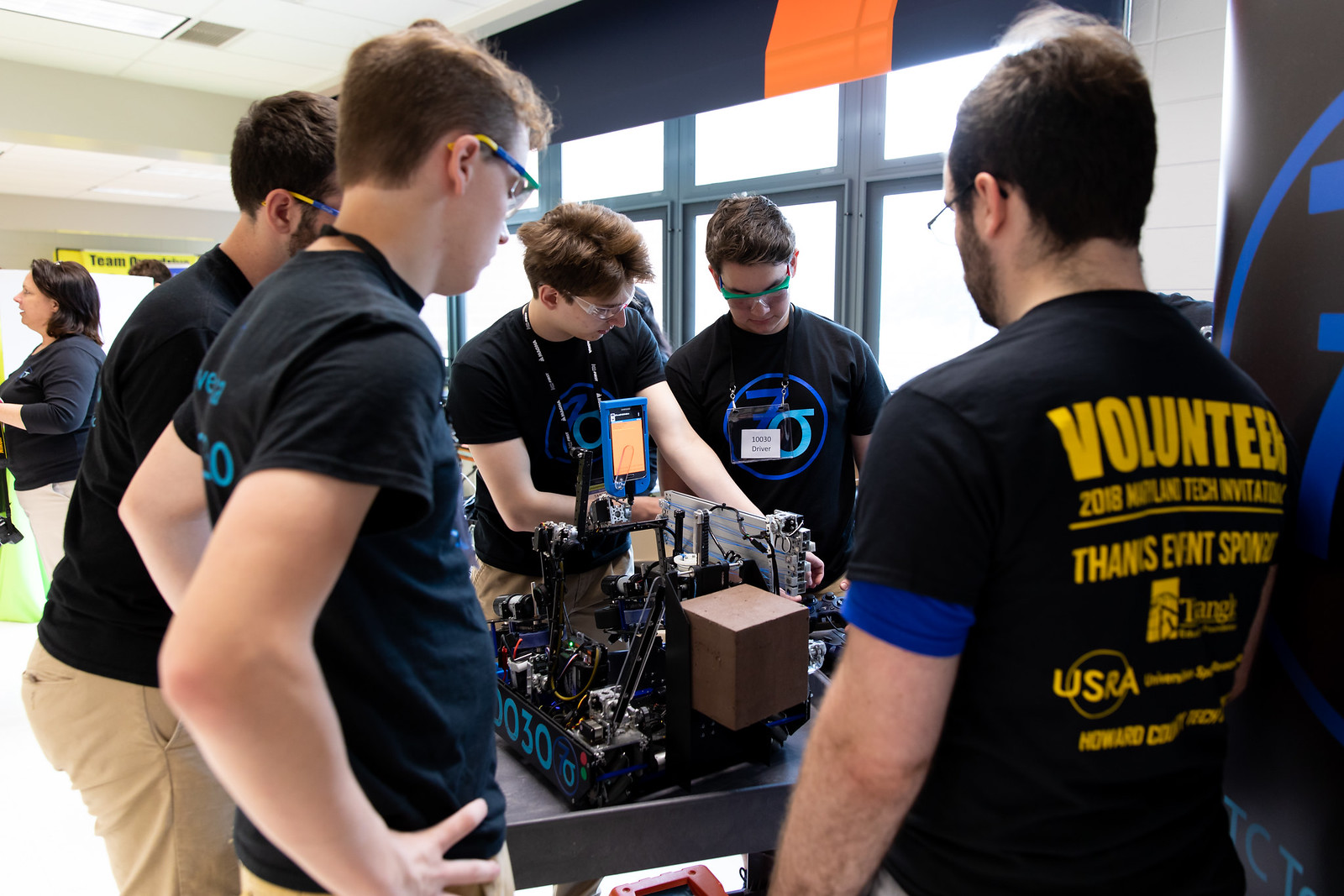The image captures six boys gathered around a table, intensely focused on a device that appears to be a robotic machine adorned with various colored components and wires, notably red, yellow, and blue. The machine features a camera and a large cardboard box on top, and a phone is connected to it. Each boy is equipped with safety glasses, giving the scene a professional, tech-savvy vibe. They are all dressed in black T-shirts, displaying a blue circular logo on the front. The back of one boy's shirt prominently reads "Volunteer, 2018 Maryland Tech Invitational, event sponsor, Tangs, USRA" in yellow text. The room is bustling with activity, with other people visible in the background, illuminated by light pouring through large windows that line the wall behind them. A significant logo, possibly a number or symbol in blue, can be seen on both their shirts and the wall to the right.